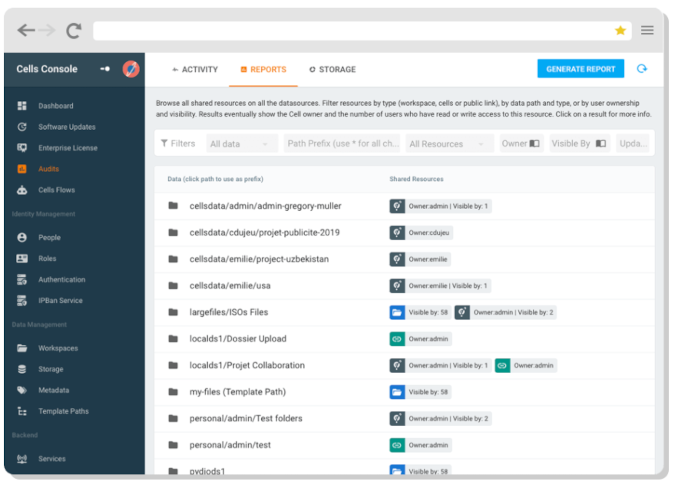This image is a screenshot from a software application called Cells Console. Dominating the top left is a Saturn-like logo featuring a blue background, a yellow ring, and an orange circle center. The image primarily displays the "Reports" section, which is highlighted with an orange background and underlined in orange. A blue "Generate Report" button is located in the upper right-hand corner of the screen.

To the left, there's a vertical menu featuring several icons and categories. The categories include:

- **Dashboard**: Overview and analytics.
- **Software Update**: System updates and patches.
- **Enterprise License**: Licensing information.
- **Audits**: Currently selected and highlighted in orange.
- **Cells Flow**: Workflow and process management.
- **Identity Management**: Subcategories such as People, Roles, Authentication, and IP Band Service.
- **Data Management**: Features Workspaces, Storage, Metadata, Templates, and Paths.
- **Backend Services**: General services.

The main pane on the right displays options to "Browse all shared resources on the data sources" and "Filter resources by type, workspace cells, or public link, by data path and type, or by user ownership and visibility." Results show detailed information about resources, like the number of users with read or write access. You can click on a result for more info.

At the top, headers allow filtering by various criteria, including "All Data," "Path Prefix," "All Resources," "Owner," "Visible By," and "Update." Listed data examples include paths like "cells data/Emily/USA" or "large files/ISOs.files."

The "Shared Resources" section to the left includes several icons representing different owners and visibility statuses, such as:
- Owner: Admin; Visible by: 1
- Owner: CDUJEU; Visible by: 58
- Owner: Admin; Visible by: 2

The icons and exact paths are mostly unreadable or unclear, with many displaying as generic placeholders or indistinct blurs.